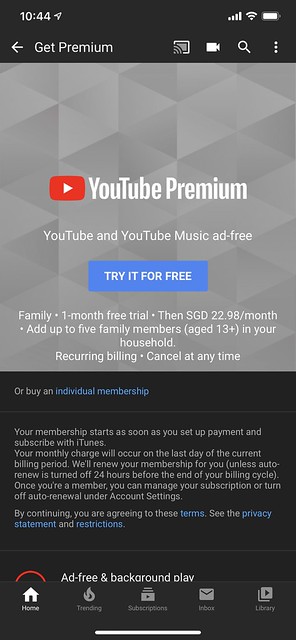Here is a detailed and cleaned-up caption for the described screenshot:

---

This screenshot showcases a smartphone screen in dark mode with a black background. In the upper left corner, the time "10:44" is displayed alongside a send icon. The upper right corner contains symbols for network connectivity, battery bar, and battery percentage.

The upper half of the screen features a geometric background of gray triangles. Prominently displayed is the YouTube Premium logo, consisting of the white text "YouTube Premium" adjacent to the red-and-white YouTube symbol. Below this, it reads "YouTube and YouTube Music ad-free." 

A blue call-to-action button beneath this text states "Try it for free" in white font. Further down, there is a description that says, "Family one month free trial then SGD 22.98/month. Add up to five family members (ages 13+) in your household. Recurring billing. Cancel at any time."

The bottom half of the screen has a solid black background. It includes an option labeled "Or buy an individual membership" in gray, followed by detailed subscription information in blue text. It states, "Your membership starts as soon as you set up payment and subscribe with iTunes. Your monthly charge will occur on the last day of the current billing period. We'll renew your membership for you (unless auto-renew is turned off 24 hours before the end of your billing cycle). Once you're a member, you can manage your subscription or turn off auto-renewal under Account Settings. By continuing, you are agreeing to these."

Highlighted in blue are the words "Terms," "Privacy Statement," and "Restrictions," with "See the" and "and" appearing in gray.

At the bottom of the screenshot, there are navigation icons for "Home," "Trending," "Subscriptions," "Inbox," and "Library," along with their respective symbols. Text indicating "Ad-free background play" accompanies these icons, along with a red upside-down semi-circle symbol.